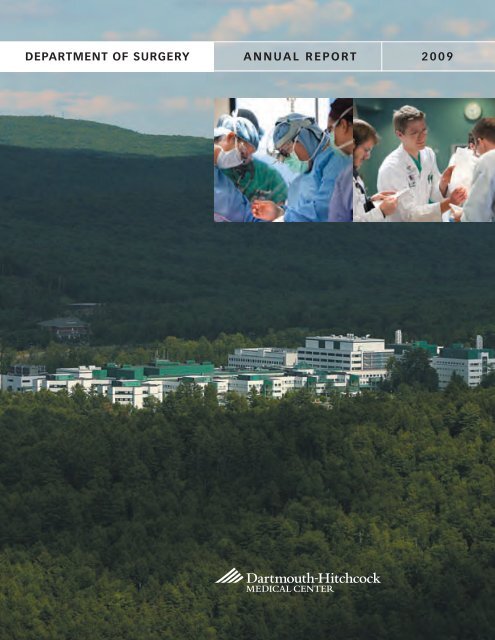The image showcases an aerial view of the Dartmouth-Hitchcock Medical Center, a significant medical complex nestled within a vast, densely wooded area with hills visible in the background. The center features a series of white buildings, interconnected and topped with flat, green-turquoise roofs. At the bottom of the image, white text reads "Dartmouth-Hitchcock Medical Center." The top portion of the image is designated for texts and divided into three sections: "Department of Surgery," "Annual Report," and "2009." Just below these headings, there are two side-by-side photographs. The first image depicts surgeons in blue surgical suits and masks, while the second shows doctors in white lab coats examining documents together.